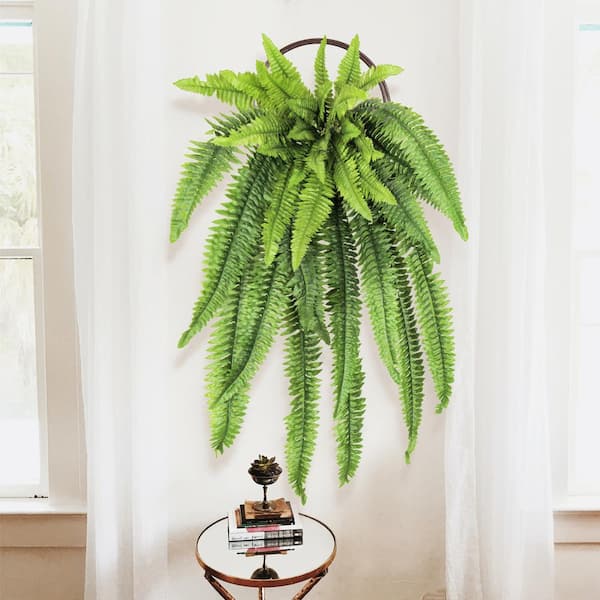This detailed vertical rectangular photograph captures the elegant interior of a living room, prominently featuring a stylish central arrangement. The focal point of the image is a lush, green fern hanging from a pot, positioned between two old-style windows with white frames and panes. Gauzy white curtains frame each window, adding a soft touch to the scene. Below the fern, a small, round table with a reflective, mirror-like surface and gold trim stands out. The table holds a neat stack of around five books and a metallic chalice, adding a touch of sophistication. The wall behind is primarily white with a beige lower section, contributing to the room's airy and inviting atmosphere.